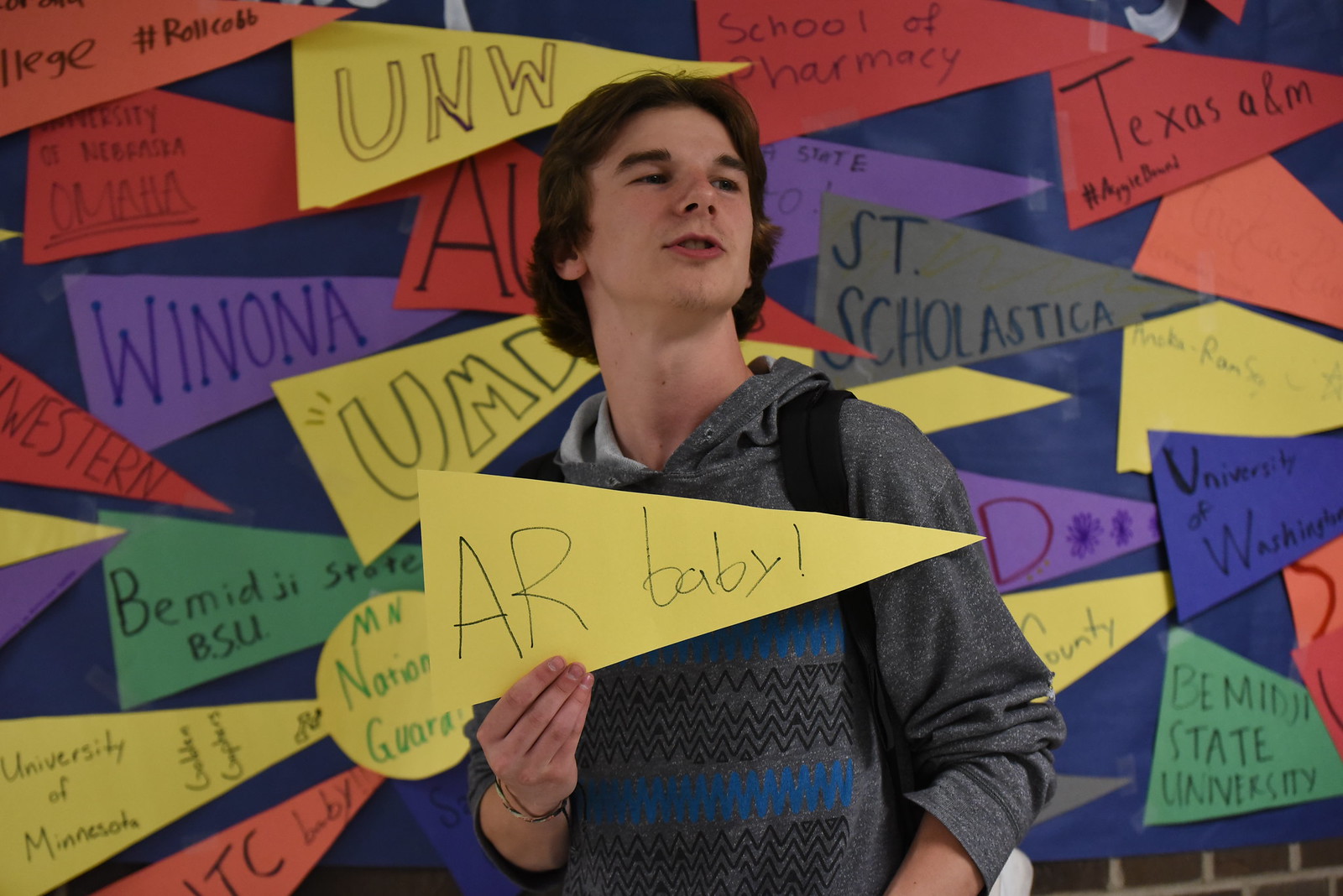The image features a young man, possibly a teenager, standing with his body facing the camera but his head slightly turned to the left. He has medium-length brown hair and is wearing a gray hoodie adorned with blue and black zigzags on the front. A black backpack strap is visible on his left shoulder. In his hands, he holds a yellow pennant with handwritten text that reads "AR BABY!" in a mix of uppercase and lowercase letters. Behind him is a vibrant, blue wall covered with numerous, colorful triangular paper pennants. These pennants display various university names, including Winona, UNW, Texas A&M, UMD, St. Scholastica, BMIJI, State University, the University of Washington, and the School of Pharmacy. The wall creates a backdrop filled with an array of colors such as red, purple, green, gray, and blue. The young man's stance and the lively background of collegiate pride convey a sense of youthful enthusiasm and academic celebration.